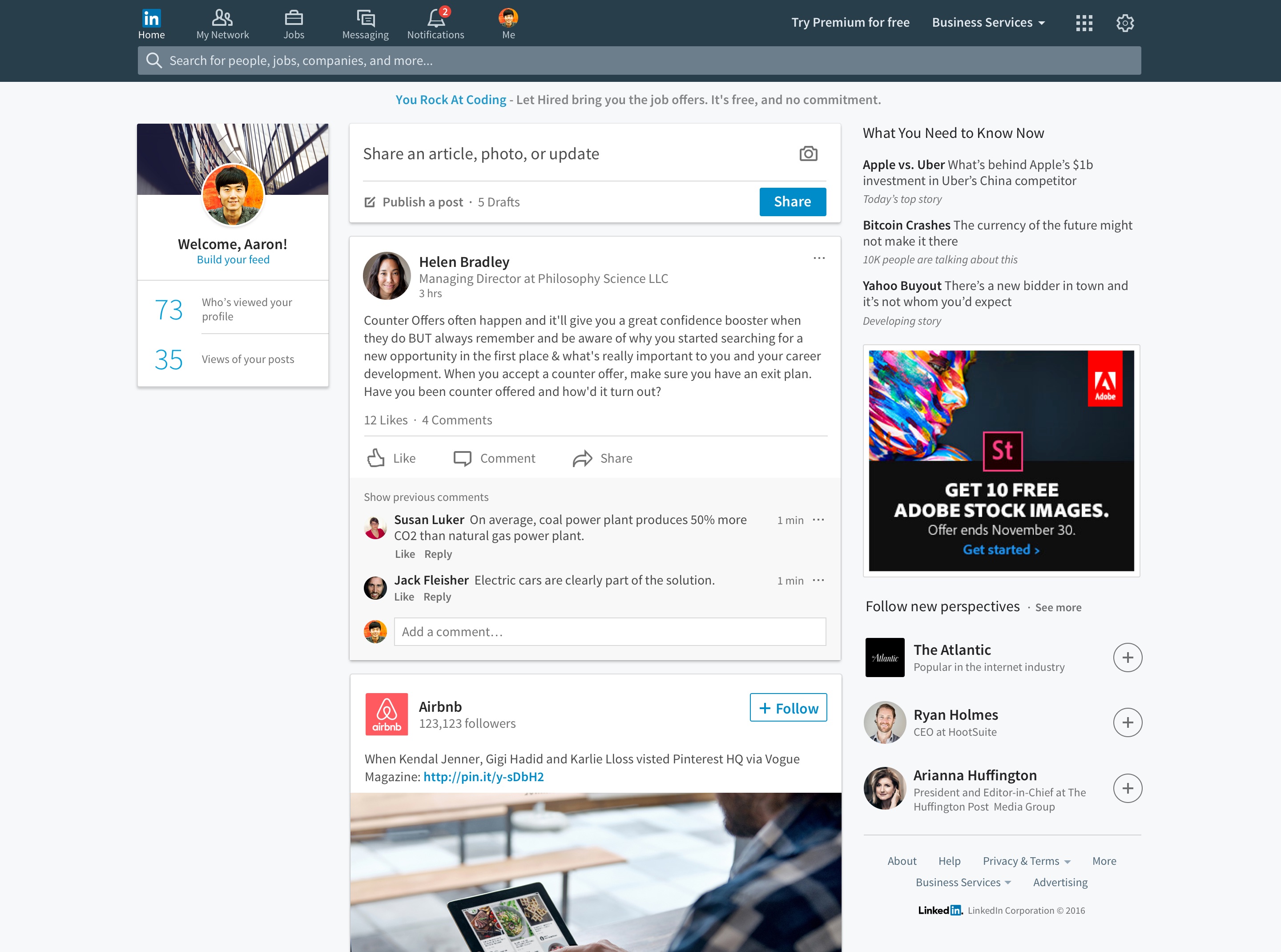This is a detailed description of a profile page on Indeed, specifically for a user named Aaron.

At the top of the page is a black banner that spans the width of the screen. Inside this banner, on the far left, is a gray search bar. Directly above it, there are navigation options including the home page for Indeed, My Network, Jobs, Messaging, Notifications, and the profile page labeled "Me." To the right, there is a button prompting users to "Try Premium for Free," followed by a drop-down menu labeled "Business Services" and a settings icon.

On the left side of the page, there is a rectangular box welcoming Aaron, which contains Aaron's profile picture. Below the picture, it shows that 73 people have viewed Aaron's profile, and 35 people have viewed his posts. At the very top of this section, in blue text, there's an encouragement saying, "You Rock at Coding. Let Hired Bring You the Job Offers. It's free and no commitment."

Further down, Aaron has the option to share an article, a photo, or an update. Below this sharing option is a post from Helen Bradley, the Managing Director at Philosophy Science, LLC. Helen’s post discusses the common occurrence of counteroffers in job negotiations, advising readers to remember their initial motivations for seeking a new opportunity and to be aware of their career development goals. She emphasizes the importance of having an exit plan when accepting a counteroffer and invites others to share their experiences with counteroffers.

The page is also populated with additional secondary content and advertisements.